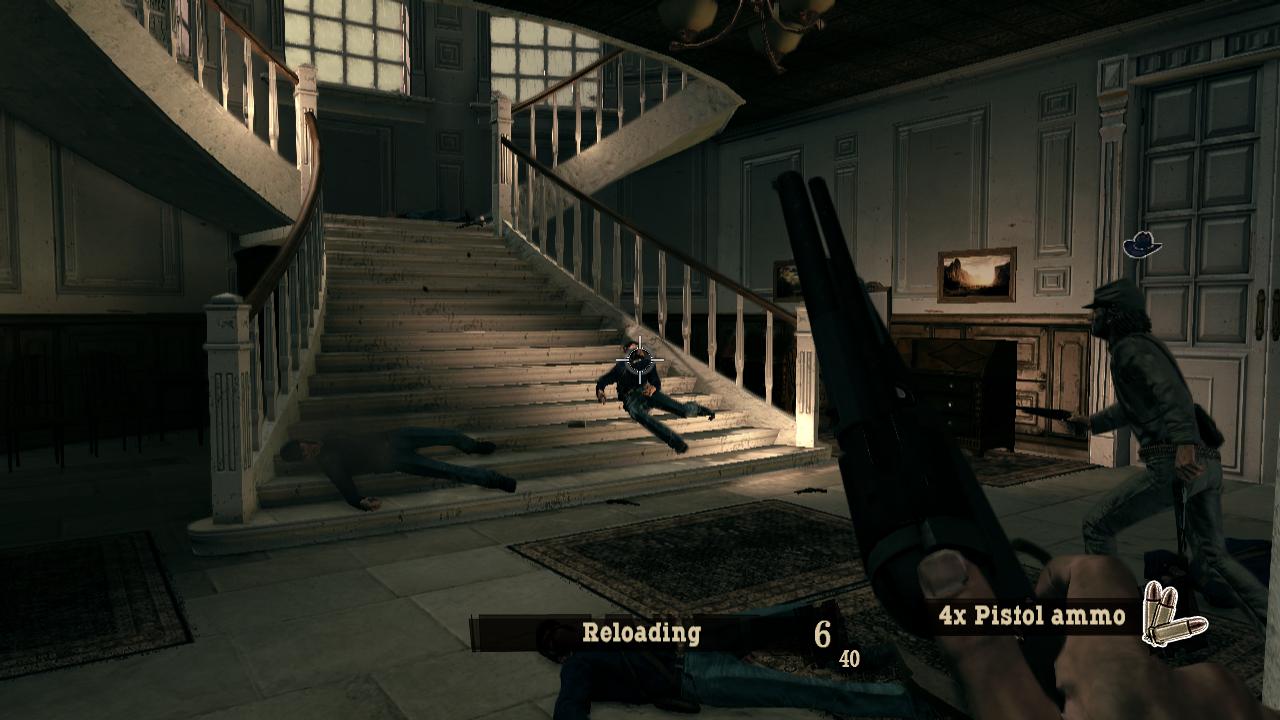A highly immersive screenshot from a historical video game captures intense action in a wealthy mansion setting. At the bottom of the screen, the game's interface displays two key status indicators: the word "Reloading" in large font with the number "6" below it, and in slightly smaller font, the number "40". To the right, "4x Pistol Ammo" appears next to a small icon depicting three bullets.

In the foreground, there is a first-person perspective of a character gripping a weapon, presumably a pistol, with the thumb and fingers clearly visible, the weapon pointed upwards. In the middle distance, a Confederate soldier dressed in typical gray attire and a sloped Civil War cap is in motion, racing towards an elaborate staircase. This staircase, indicative of a mansion's opulent interior, features a lush Persian rug at its base.

On the stairs, two distressed figures are visible: one body is sprawled out across the lower steps, while another person appears to be collapsing, possibly clutching their abdomen in pain. Crosshairs target the second figure's head, adding to the tension of the moment. Above the Confederate soldier, a small cowboy hat icon lingers, providing an additional layer of intrigue to the already dramatic scene.